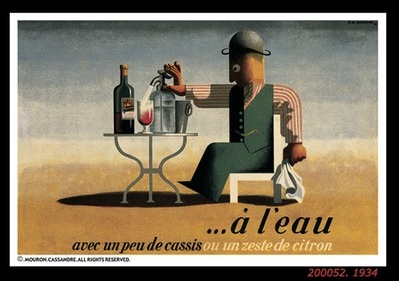The image in question is a detailed, colored drawing that appears to be a postcard, lithograph, or print, possibly created by Jacobin Cassandre, as indicated by the artist and copyright information, with a number, 200052,1934, suggesting it might be a limited edition. It features a scene with a man seated on a white chair on the right side, framed in black. He wears a distinctive outfit consisting of a red-and-white striped shirt, a black vest, and black pants. The man is positioned at a small, three-legged table with curved legs, topped with various items: a glass full of red liquid, a bottle of wine, a dispenser pouring liquid into the glass, and a bucket. The background suggests an outdoor setting with a blue sky and a sandy floor. Additionally, below the image, some text in foreign languages is visible, including the phrases "aloo" in black and "oo on zest de citron" in white.